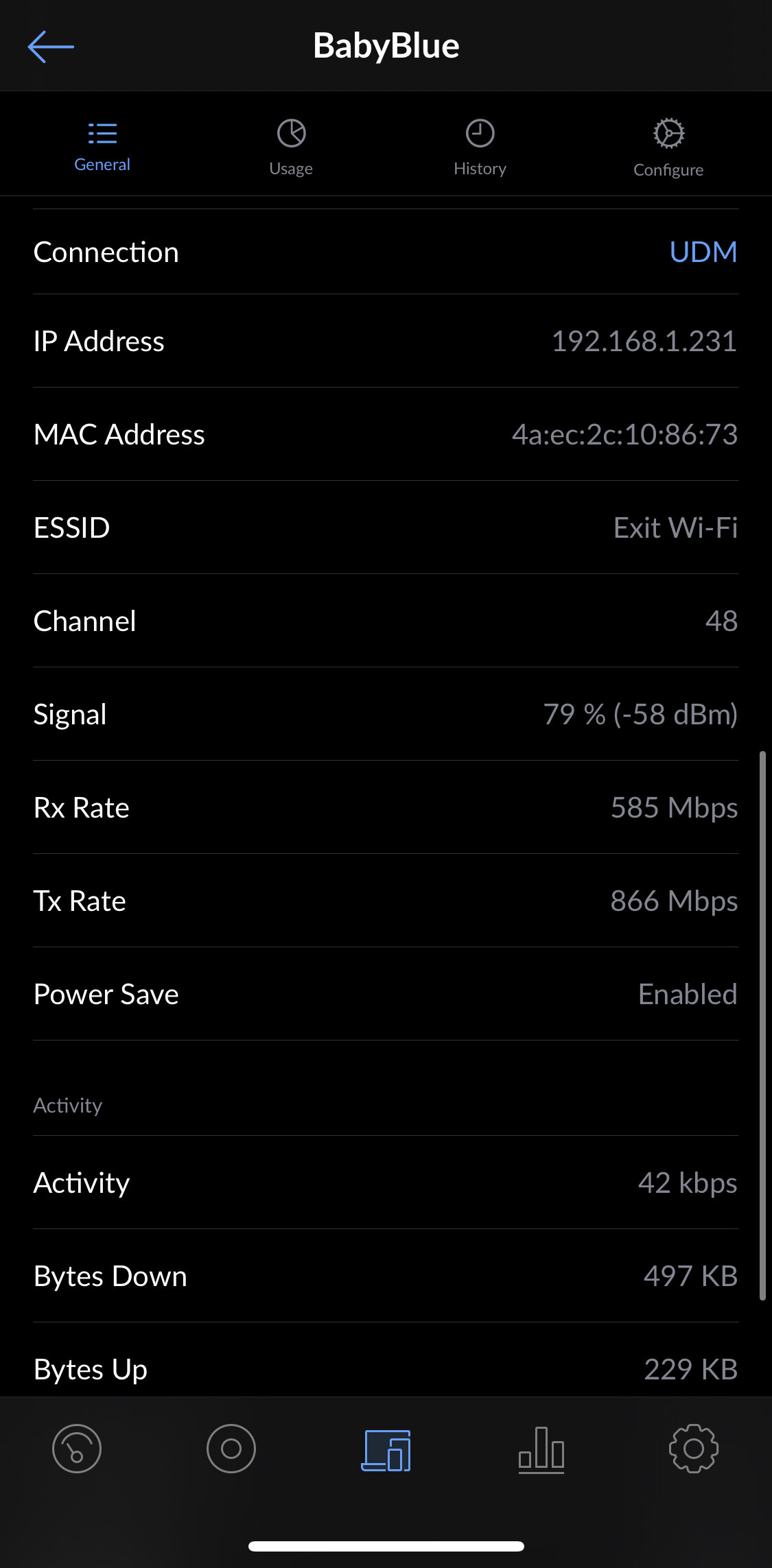In this image:

- The backdrop is a black background.
- A left-pointing blue arrow, along with a baby blue section, is prominently displayed.
- Various labeled sections are visible, including "General Usage," "History," "Configure," and "Connection."
- Device information is detailed, such as:
  - IP Address: 192.168.1.231
  - MAC Address: 4AAC2C10A673
  - ESSID: Wi-Fi
  - Channel: 48
  - Signal Strength: 79% (-58 dBm)
  - RX Rate: 585 Mbps
  - TX Rate: 866 Mbps
  - Power Save: Enabled
  - Activity: 42 Kbps
  - Bytes Down: 497 Kbps
  - Bytes Up: 229 Kbps
- On the interface, a circular icon resembling the dawn symbol is present.
- Device icons for a laptop, smartphone, and tablet are visible.
- A graph is displayed within the interface.
- A grey gear icon, representing settings, is situated at the bottom of the image.
- A horizontal white line separates elements towards the bottom.
- A scroll bar is located on the right side of the image.

This detailed snapshot provides comprehensive information about the connected network device and associated data metrics.